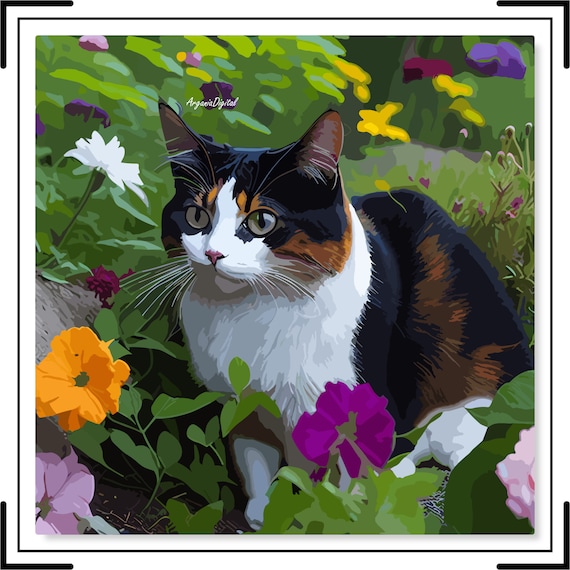This image is a digital painting that features a calico cat with striking details. The cat's fur is predominantly black, with a white chest, mouth, and foreleg, and orange highlights adorning its face and running down its side. Its eyes have a captivating greenish hue surrounding the black pupils, and the nose is a delicate pink. The scene is set outdoors in a garden, where the cat sits amidst a lush array of green leaves and colorful flowers; pink, orange, purple, and white blossoms are scattered around it. Behind the cat, the background is filled with tall grass and blurred flowers, adding depth to the setting. A small, hard-to-read signature, possibly 'Aranea Digital,' is located above the cat. The entire painting is bordered in white with black L-bracket lines at each corner, framing this serene moment.